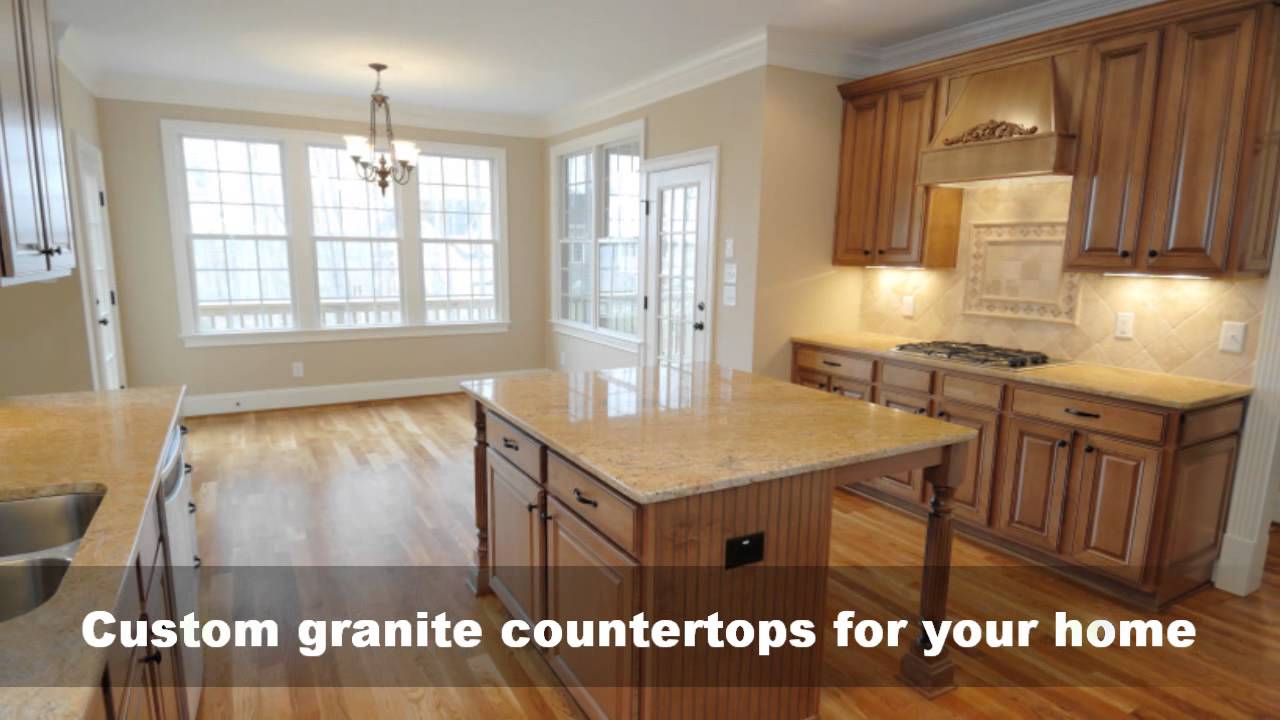This rectangular photograph, likely intended for an advertisement, showcases a beautifully remodeled, spacious kitchen bathed in natural light. The focal point is an elegant granite center island, with matching honey-colored granite countertops surrounding it. Medium brown wooden cabinets with black handles frame the kitchen, while a hardwood floor extends throughout the room. To the left of the island, an expansive countertop houses a sink, and to the right, another granite surface includes a stovetop. The room features large windows on the far wall and to the right, along with a French door and a small chandelier above, suggesting a designated dining area. Superimposed at the bottom, white text reads: "Custom granite countertops for your home," underscoring the kitchen's gleaming stone surfaces. The space appears meticulously staged, reminiscent of a model home, hinting at an ideal setting filled with potential and contemporary elegance.